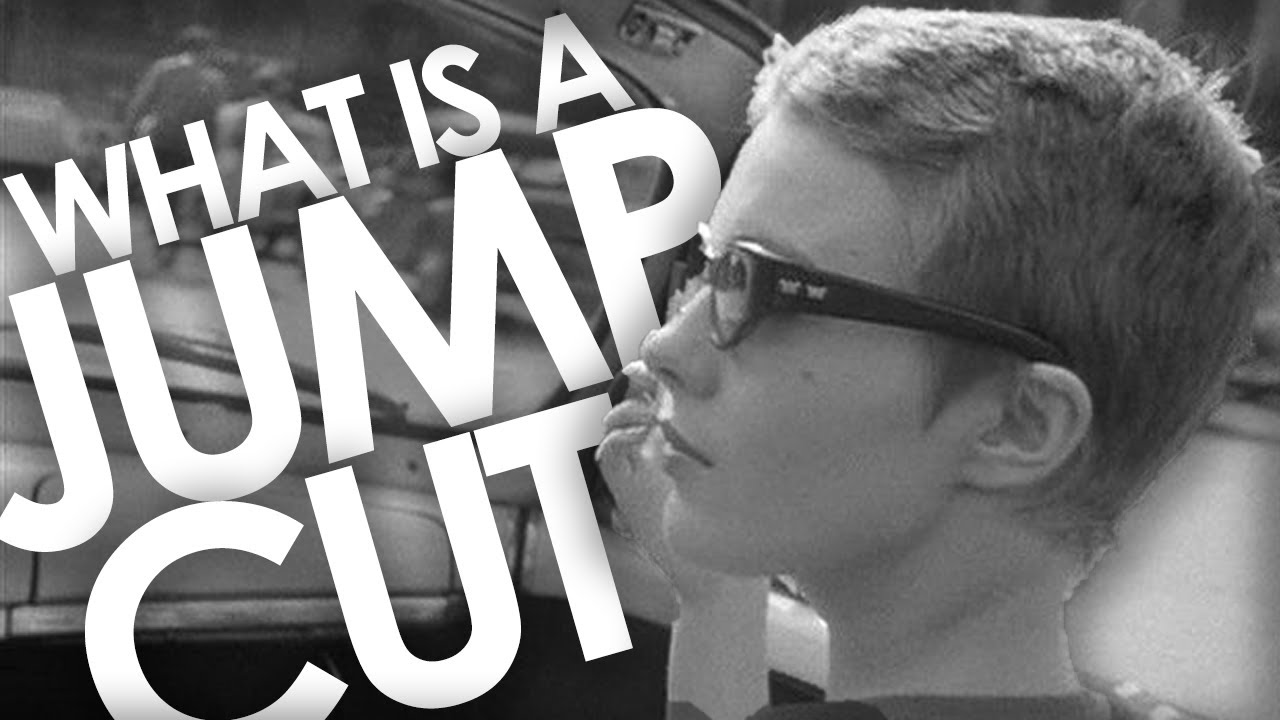This black and white photograph captures a close-up side profile of a teenage boy, approximately 15 years old, who is seated in the passenger seat of a convertible car with the top down. The boy, gazing leftward, is dressed in black sunglasses and has a short haircut, with his closed mouth giving a neutral expression. Superimposed across the image in large, bold white text are the words "What is a jump cut?" suggesting the image may be related to teaching film editing techniques or could be an advertisement for a salon. In the blurred background, a couple walks down the sidewalk, and multiple cars populate what appears to be a street or parking lot scene. The overall composition includes visible elements of the car such as the windshield and wipers, adding to the contextual ambiance.